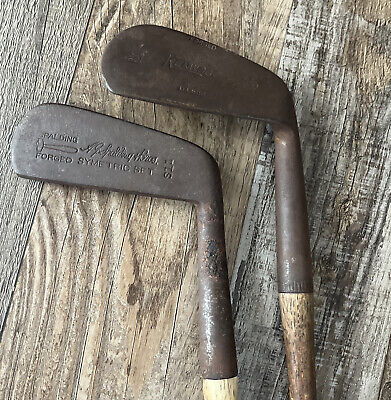This professional portrait photograph features two antique golf clubs, likely putters, positioned side by side on weathered, light-colored wooden surface. The club heads are dark, rusted, and corroded, accentuating their age and frequent use. Each club head bears inscriptions; the more legible bottom club reads "Spalding Forged Symmetric Set" with additional faint cursive script and a number that resembles "S11." The text on the top club is much fainter and nearly impossible to decipher. The worn wooden shafts extend slightly from the heads, maintaining the aged theme of the objects, creating a striking contrast between the dark corrosion of the metal and the lighter wood.